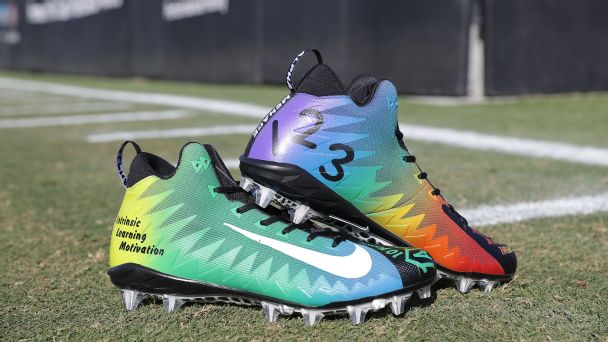This image showcases a pair of vibrant Nike cleats, likely designed for soccer but possibly adapted for other grass sports such as lacrosse or rugby. The close-up side view highlights two stacked cleats, featuring a mix of colors in a tie-dye, rainbow-like pattern. Both shoes display a distinctive white Nike swoosh. The bottom cleat is predominantly green and blue with black laces and the words "learning and motivation" inscribed near the heel. The top cleat flaunts hues of blue, yellow, orange, and red with the numbers "1, 2, 3" in black. The cleats rest on a sports field with grayish-green grass and white chalk lines, indicative of game markings, with a blurred black perimeter fence visible in the background. The overall setting emphasizes the dynamic and motivational theme of the cleats.